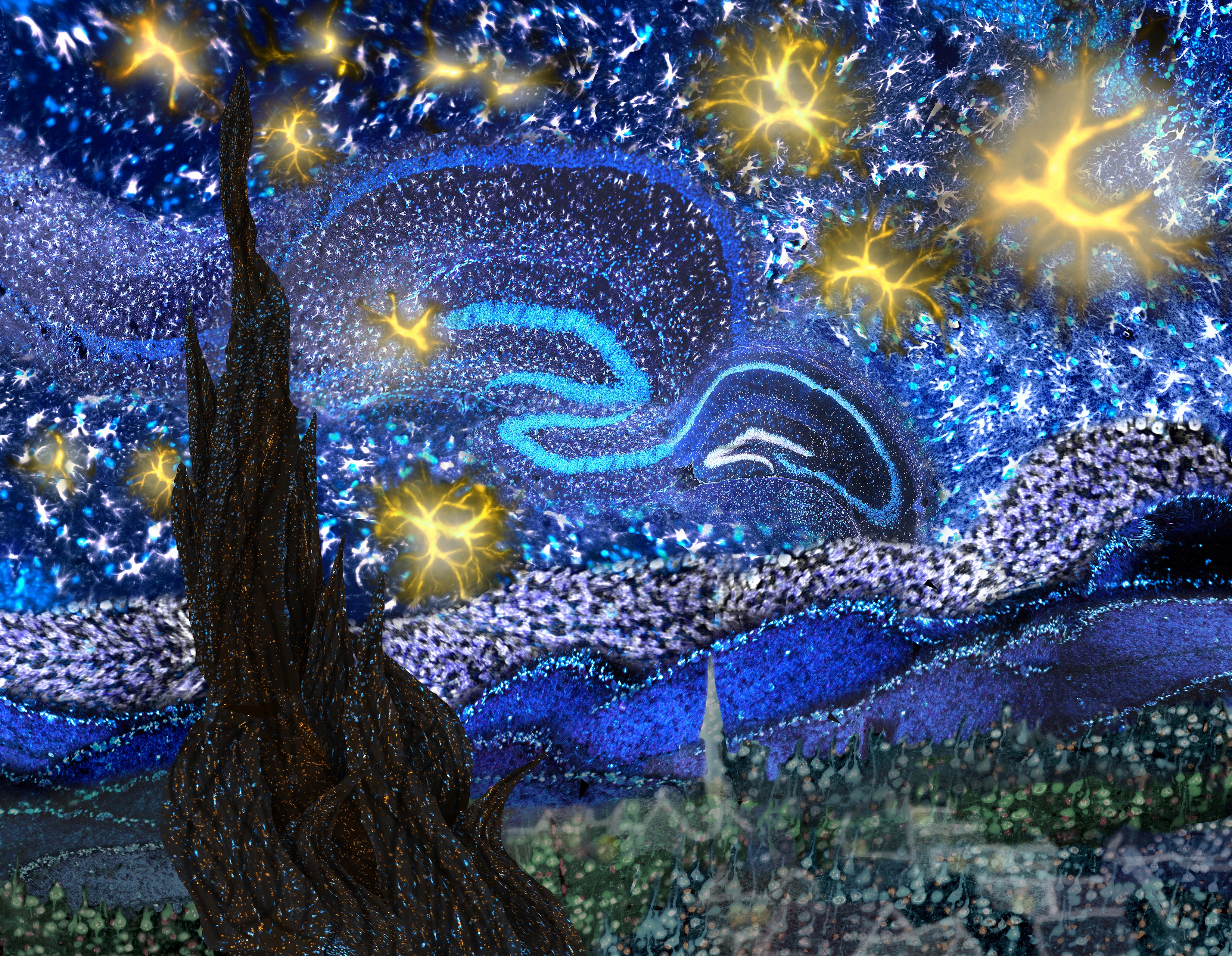The image appears to be a digital or painted artwork inspired by Van Gogh's "Starry Night," with a distinct emphasis on tree motifs. At the center front, there's a gnarled, leafless tree trunk, dark brown and embedded with blue sparkles. The sky, predominantly dark and light blue with white swirls, is dotted with intricate, yellow, and gold patterns resembling electrical or lightning bolts, as well as tiny white and black dots that reinforce the starry motif. These yellow patterns are abstract tree-like fragments, replacing the traditional celestial bodies seen in Van Gogh's work. The bottom section of the image showcases green foliage, rolling blue hills, and hints of water in grays and blues. The left side features a tall, dark plant that oversees a distant town in the bottom right, adding depth and grounding to the busy composition. This artwork, possibly utilizing pointillism, is richly detailed with countless tiny dots creating a textured, dynamic scene that intricately blends natural and celestial elements.